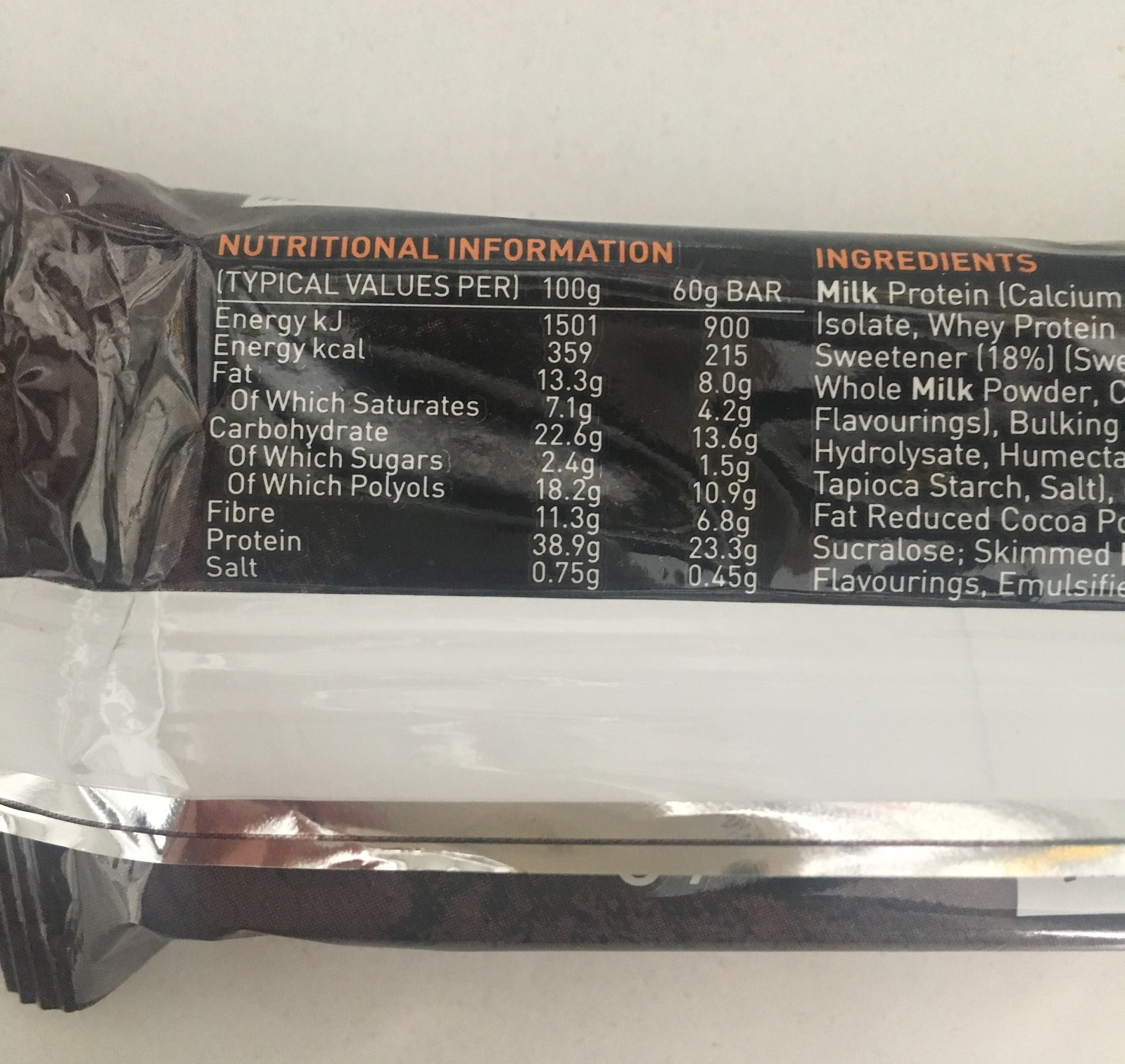The image displays the backside of a black plastic food packaging, specifically an energy bar. The focal point is a prominent white strip near the bottom, stretching from left to right. Visible on the left edge is a partial tag, just on screen. The packaging showcases nutritional information and ingredients in a zoomed-in view, partially off-screen to the right. This information is presented in bold orange font, while the text detailing the nutritional values like calories, fat, carbohydrates, fiber, protein, and salt is in white. The words "typical values per" followed by specific amounts and "per bar" are also visible. In addition, the packaging highlights ingredients such as protein and whey powder. A silver border can be seen on the loose edge of the bar that is positioned at the bottom, which is on its side, while the other bar lays flat on its back. The packaging background alternates between black and a light gray gradient, providing contrast to the text.